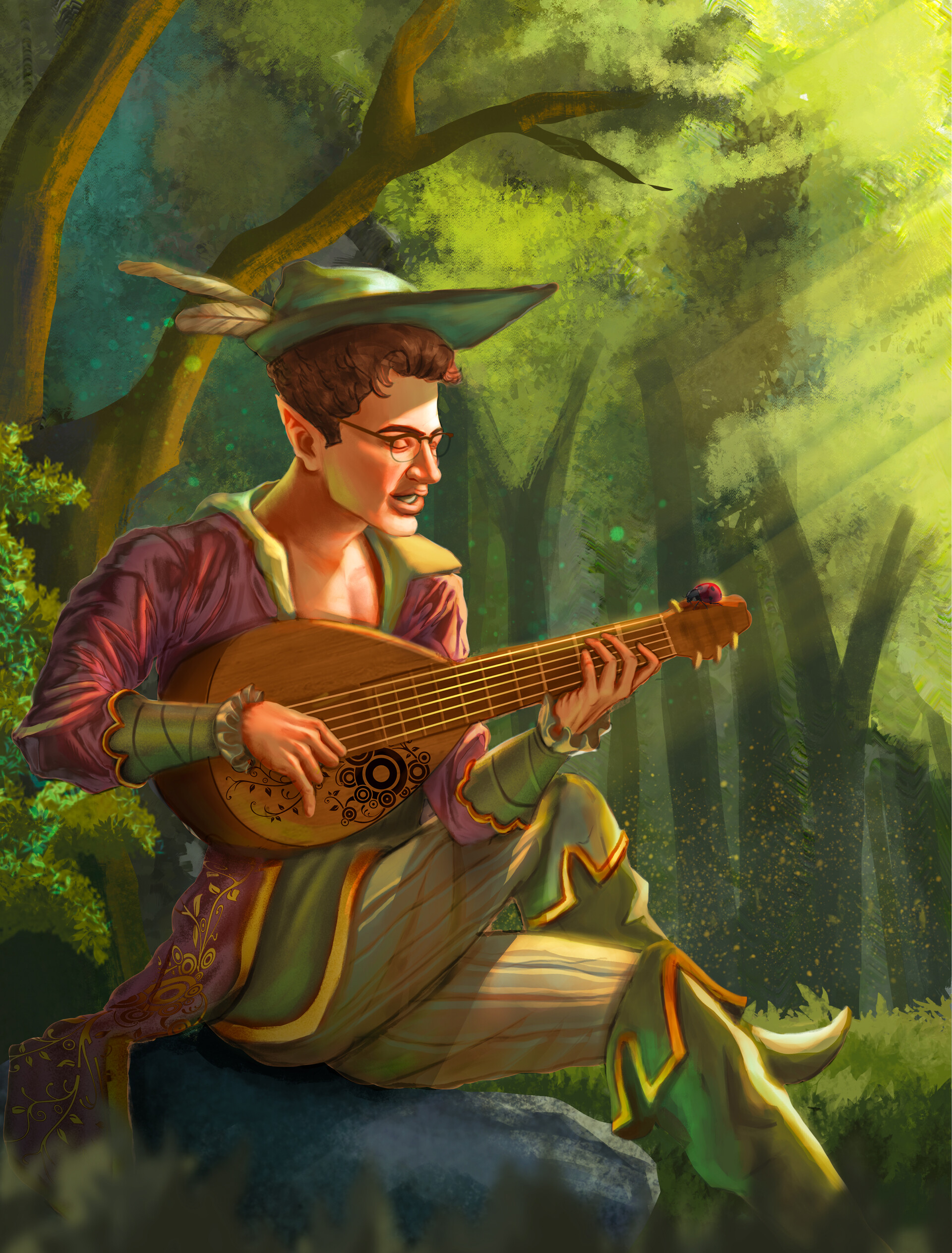In this detailed digital painting, a young male figure with elf-like pointy ears is depicted sitting in a forest, playing a lute. His eyes are closed and mouth slightly open, suggesting he is singing while strumming the instrument. This modern-day bard, envisioned in a medieval setting, wears prescription glasses that add a contemporary twist to his otherwise historical attire. He dons a pointed green hat, reminiscent of Robin Hood's, adorned with a couple of feathers jutting from the back. His outfit consists of a reddish-purple jacket over green sleeves and white-and-green striped knee-length breeches. Tall green boots with yellow trim reach up to his knees. The bard is seated on a blue rock, surrounded by a canopy of foliage from the trees behind him. Rays of light stream through the leaves, casting a serene and magical atmosphere over the scene.